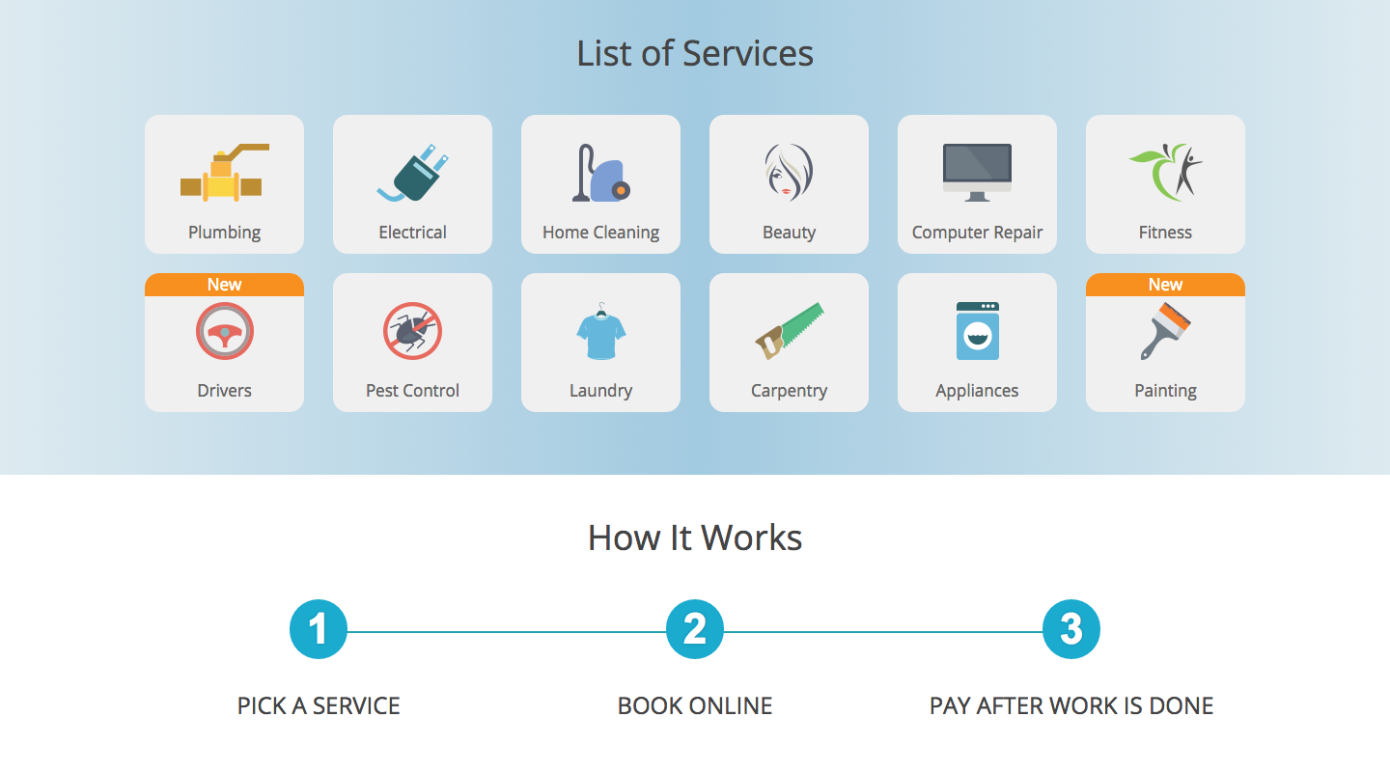In the image, a grid of service categories is presented in a structured layout. Dominating the top middle of the image is the title "List of Services" displayed in bold black text. The background transitions from a light bluish hue in the center to a cloudier, whitish color towards the far left and right edges, creating a soft gradient effect.

Beneath the title, there are two rows of six service categories, each housed within a box with a whitish gray background. 

In the first row:
1. The box on the far left is labeled "Plumbing" and features an icon of a faucet above the text.
2. Next, the "Electrical" box displays an electrical plug icon.
3. The third box, titled "Home Cleaning," shows an image resembling a lamp.
4. The "Beauty" category follows, adorned with an illustration of a woman's silhouette.
5. The fifth box reads "Computer Repair" and includes an icon of a computer monitor.
6. The last box in the first row is "Fitness," featuring an image of a person jumping in the air.

In the second row:
1. The first box is titled "Drivers," with an icon of a steering wheel and the word "NEW" prominently displayed at the top.
2. Next, "Pest Control" is depicted with an associated icon.
3. The "Laundry" box follows with a relevant image.
4. To the right, "Carpentry" is represented by an appropriate icon.
5. The "Appliance" box is next in line, depicting related imagery.
6. The final box in this row is "Painting," also marked with the word "NEW" and a suitable icon.

This detailed and organized display ensures each service category is distinctly represented for easy identification.